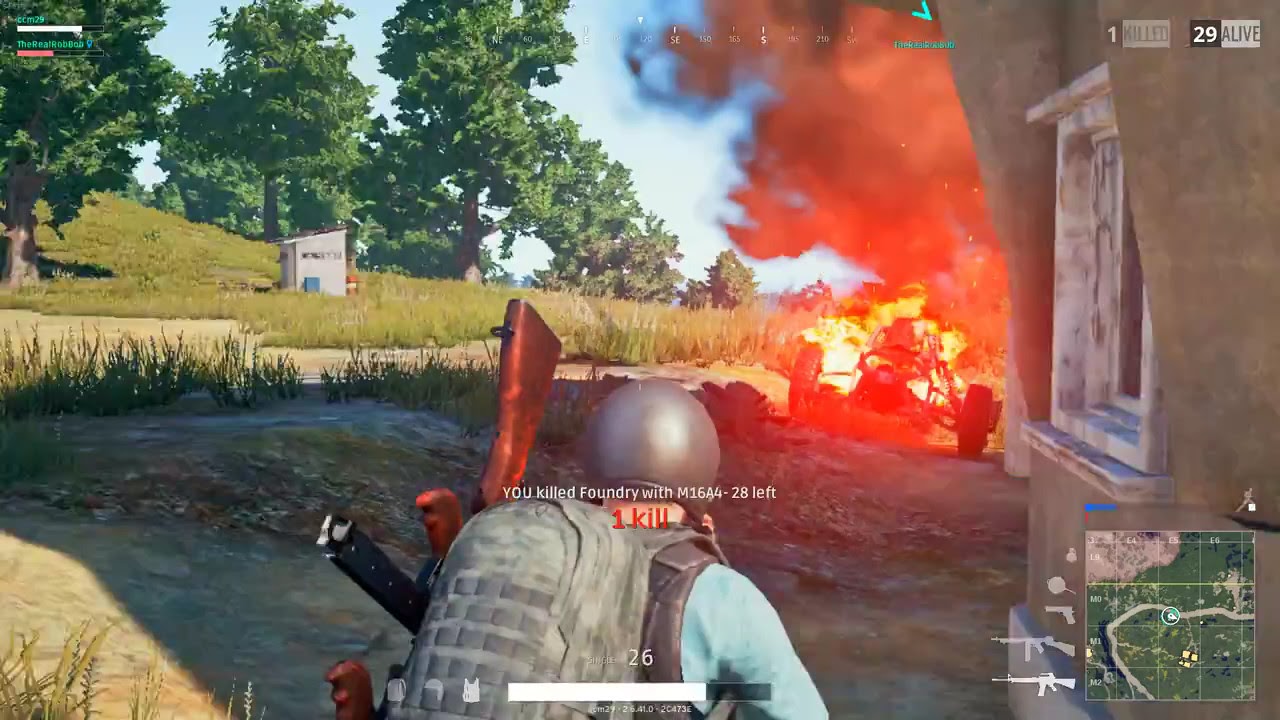This is a detailed image from a first-person shooter video game, likely Call of Duty. The main subject is a soldier viewed from behind, dressed in military attire that includes a dark silver helmet and a gray backpack. The soldier is holding an old-fashioned rifle, likely an M16A4, with a wooden stock and handle, slung over his shoulder. He is depicted sneaking around an older concrete building with a white window, which is part of a larger war-torn setting.

To the right of the soldier, there is a dramatic fiery explosion engulfing a vehicle of older design, with thick smoke rising into the blue sky. The background shows a mix of green trees and a grassy field. Notably, on-screen text indicates in white: "You killed Foundry with M16A4-28 left," and below in red: "One kill." Further game interface elements include a health bar at the bottom, showing the number 26, and a map with green coordinates in the bottom right corner.

In the upper left corner of the image, the screen name "The real Bob Bob" is displayed, likely indicating the player's identity.